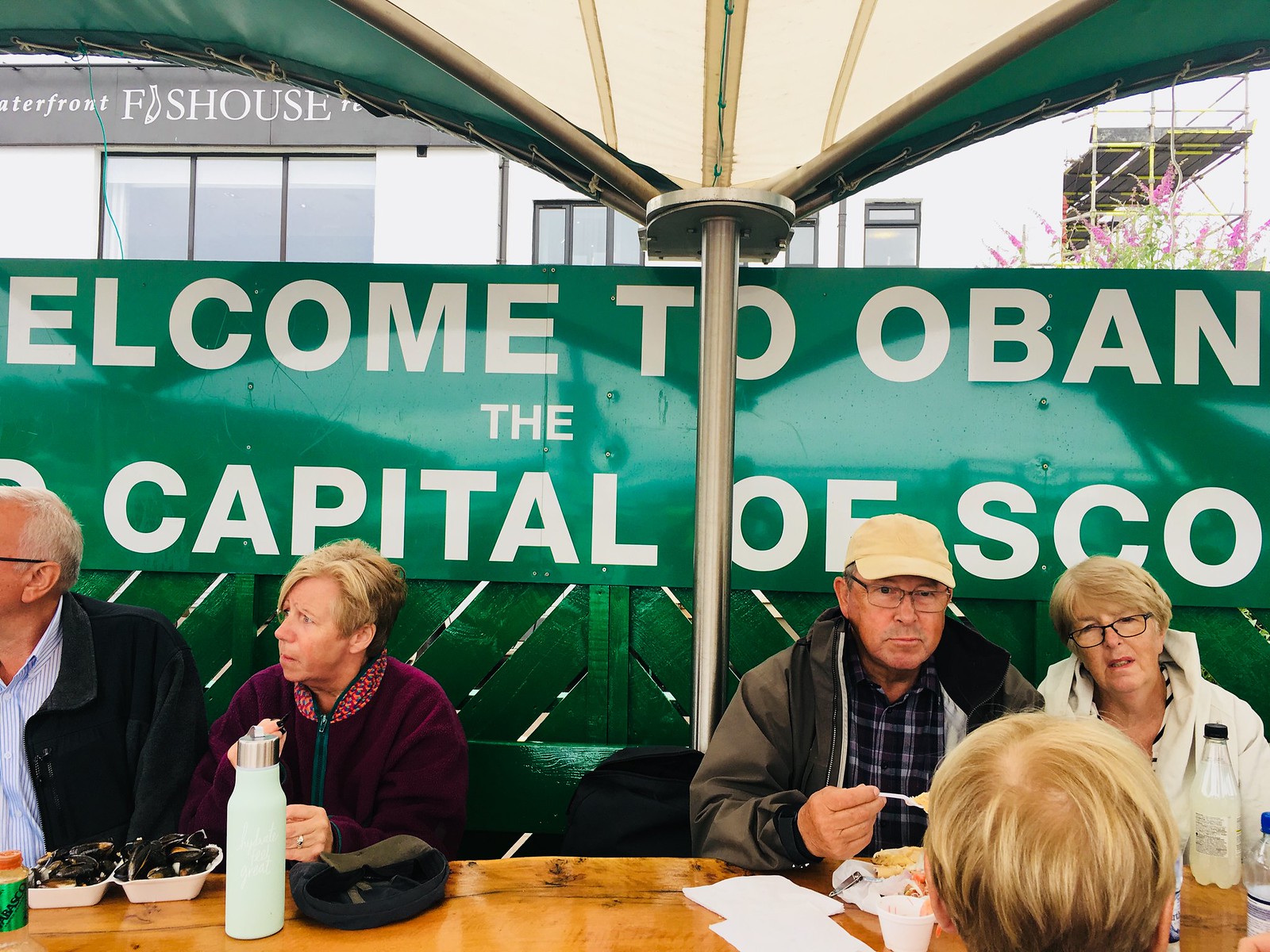The photograph captures five people dining at a brown table outside a restaurant. They sit under a large green and white umbrella on a sunny but overcast day, suggesting it might be spring with a nearby tree or bush in bloom with pink flowers. Behind them is a partially visible green and white banner that reads "Welcome to Oban, the capital of SCO," next to another sign that says "Waterfront Fish House Restaurant," where the "I" in "Fish" is creatively designed as an upside-down fish.

At the table, the group is enjoying their meal, with visible containers of mussels, cups, napkins, and a water bottle. On the right, a man wearing a white hat, a blue checkered shirt, and a brown jacket is eating, with a woman in a white jacket with blonde hair beside him. To their left, another couple sits, with the man in a black jacket, striped shirt, and glasses, next to a woman in a burgundy jacket. Additionally, the back of another blonde woman's head is visible in the foreground. The fence behind them, the pole supporting the umbrella, and some other roofing elements are all green and white, complementing the overall color scheme.